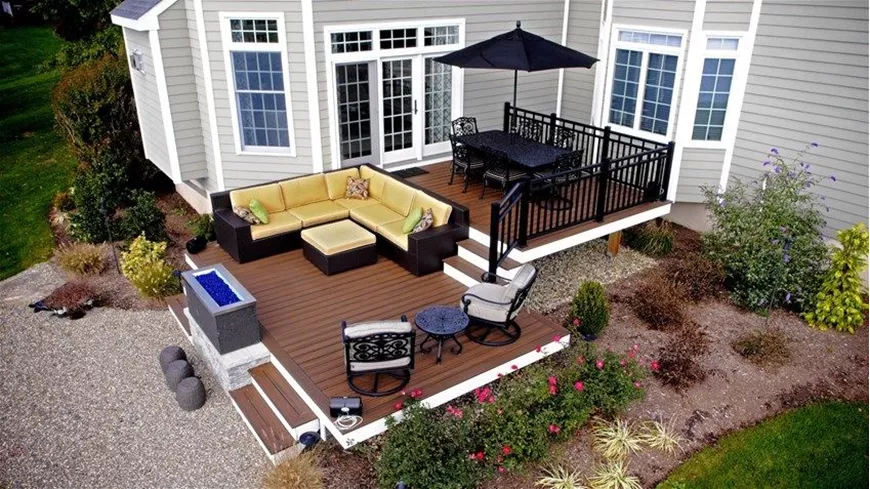The photograph showcases a multi-level patio area of a house, featuring a brown wooden porch accompanied by various outdoor furniture. The upper level of the patio includes a black dining table with a matching black umbrella, situated on a wooden deck. Adjacent to it is a small garden area with vibrant pink flowers. Descending three steps from the dining area leads to a lower level that serves as a living space, furnished with a large L-shaped outdoor sofa, two cushioned one-seat chairs, and a table. The area also includes an ambiguous blue object and a brick structure that may serve as a barbecue. Despite the detailed setup, it's notable that the patio lacks a safety fence, posing a risk of falling into the bushes below. The scene is adorned with various colors, including shades of pink, light green, yellow, black, white, gray, blue, and grassy green, blending harmoniously to create a cozy outdoor setting.